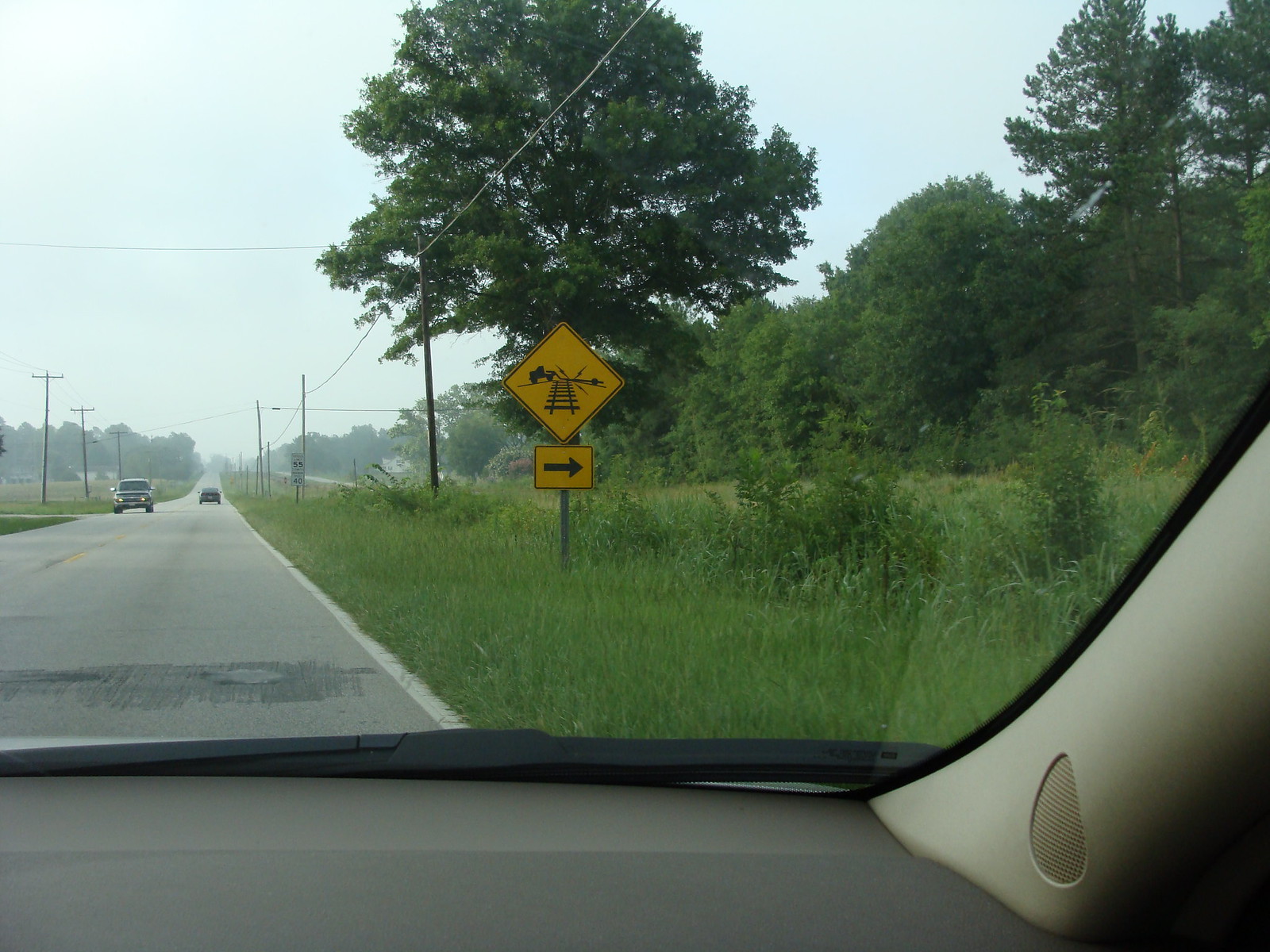In this slightly rectangular, horizontally-oriented image taken under natural overcast lighting, the viewer's perspective is angled outward from the passenger side windshield. Positioned on a two-lane road, the left side of the frame shows the road stretching into the distance, appearing narrower as it recedes. A truck is seen approaching in the opposite lane, and a car is visible far ahead in our lane.

On the right side of the frame, tall grass dominates the shoulder, gradually giving way to a dense line of large, full, green trees further to the right. Amidst this high grass, two traffic signs stand out: The top sign is a yellow diamond tilted so that its corners point up and down, displaying an image of a railroad track intersecting a road with a small vehicle crossing it. Below this is a smaller, horizontally rectangular yellow sign with a black border, featuring a black arrow pointing to the right.